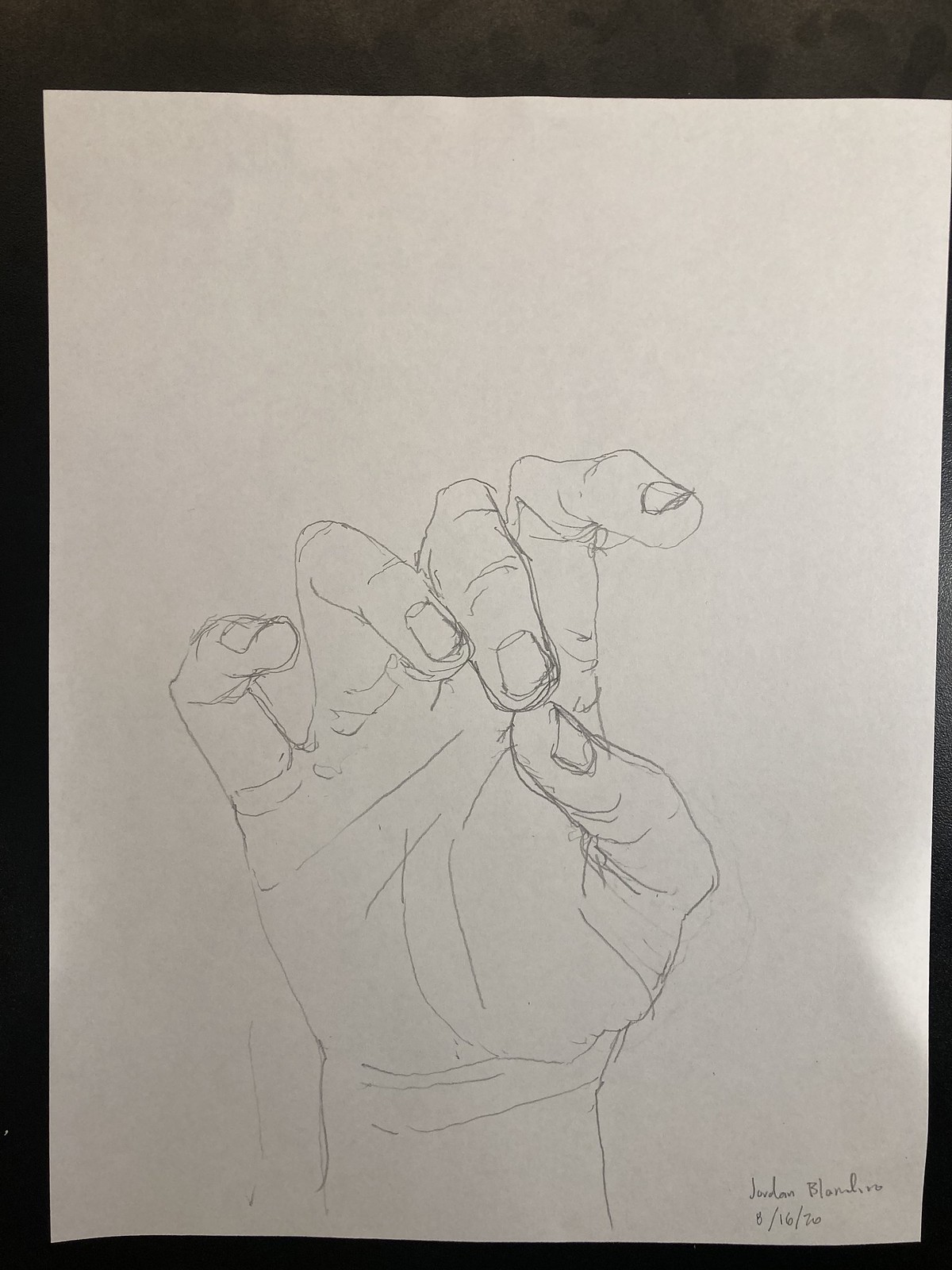This is a detailed pencil drawing of a right hand, prominently displayed on off-white paper. The hand is oriented palm-down and positioned towards the front, with the thumb and middle finger touching. The bent fingers expose the nails, adding a realistic touch to the sketch. Fine lines detail the contours and creases of the hand, enhancing its life-like appearance. The thumbnail is particularly visible and forms a central element in the lower portion of the drawing. The artist has signed the work in the lower right-hand corner, and it is dated 8/16/20. The drawing is photographed against a stark black background, which contrasts sharply with the off-white paper, making the hand drawing stand out even more intensely.